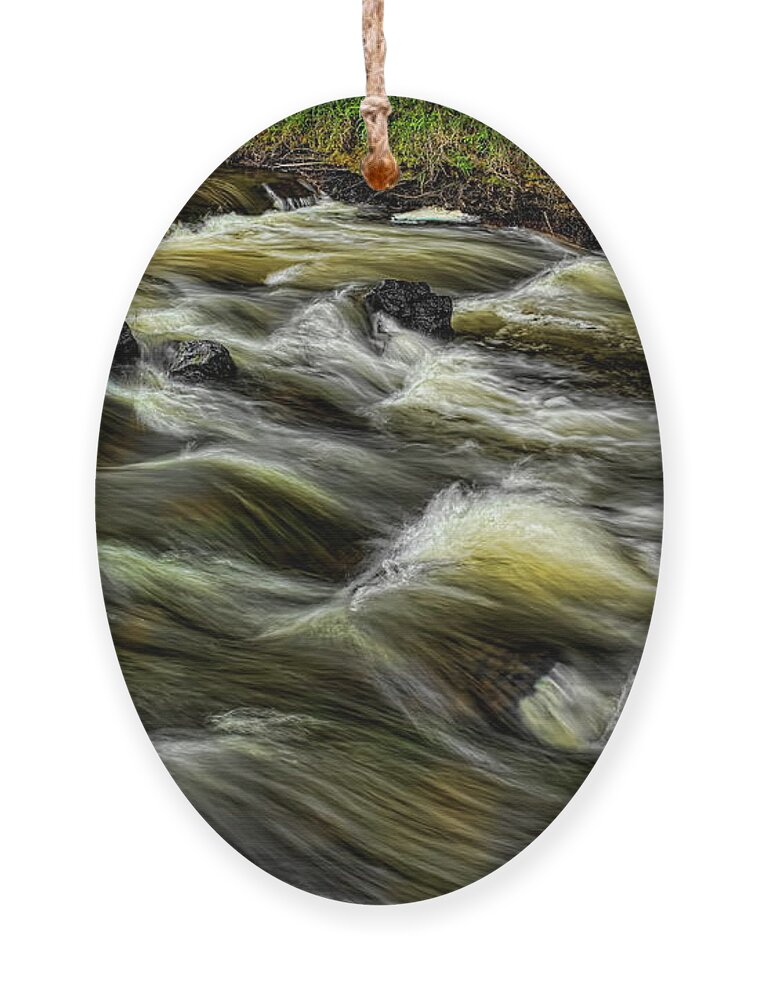This photograph depicts an oval-shaped pendant with a painting or print of a rapidly rushing river. The oval pendant has a small hole at the top, from which a piece of rope or string is tied, suggesting it's designed as a necklace or medallion. The artwork on the pendant vividly captures a gushing river with fast-moving waters characterized by white caps, indicative of turbulent rapids. The water itself is a dark, greenish-brown color, rushing violently over gray and black rocks. Along the riverbank, which is visible at the top edge of the pendant, there is dark brown or blackish dirt interspersed with green grass and some brown plants. The background of the photograph is plain white, emphasizing the pendant. The painting on the pendant might give an illusion of depth and movement, almost resembling hair with its flowing patterns. This detailed depiction not only shows the intensity of the flowing water but also hints at elements of nature like rocks and vegetation, captured in a small, oval frame.